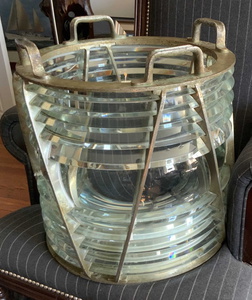The photograph features a cylindrical, semi-transparent ice bucket placed on a dark blue single-seater sofa adorned with white parallel lines. The main body of the bucket is made of glass, which has multiple circular segments or layers, creating a textured, grasp-friendly design. It is encased in a gold-bronze metallic frame that includes four handles at the top for easy transport. The metallic structure appears slightly rusty but maintains its brass-like color. This setup is positioned in an indoor setting with a brown wooden floor visible in the background. The lighting highlights multiple reflections on the glass surfaces, adding to the intricate details of the arrangement. The entire scene suggests a blend of functionality and aesthetic charm, evoking curiosity about the ice bucket's purpose and history.